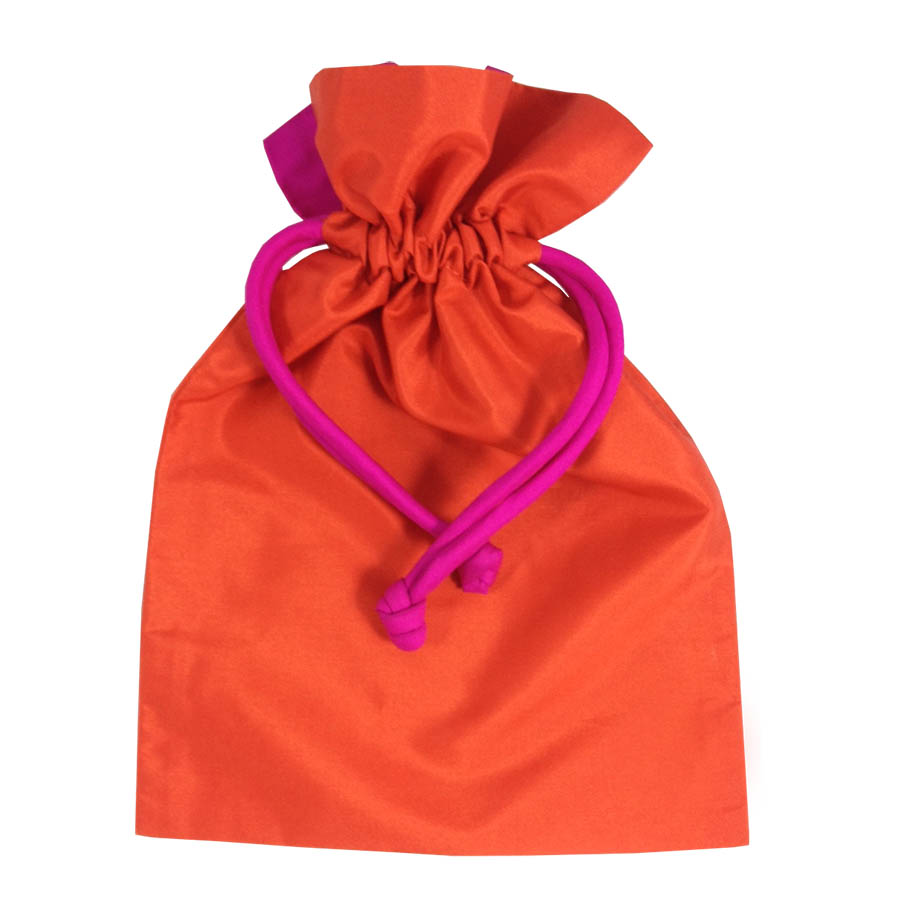This close-up photograph showcases a small, delicate drawstring pouch, primarily orange in hue with a faint sheen that suggests a slightly satin texture. The fabric appears lightweight and flexible, forming a flat, square shape that indicates the bag is empty. The drawstring, comprising two bright pink cords knotted together, cinches the top shut with the cords extending towards the center, lying over one another and creating almost a heart shape. These cords are notable for their vibrancy and the wrinkles where they gather the fabric of the pouch. The background of the image is a stark, featureless white, giving an impression of the pouch being isolated, possibly via photo editing, enhancing the focus on its modest yet colorful appearance.